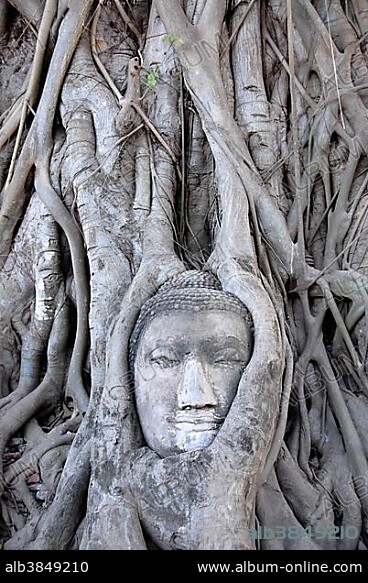The photograph showcases a striking close-up of intricately intertwined tree roots enveloping a stone-carved face, seemingly that of a woman with hair styled in a bun. This natural-artistic fusion gives the impression the face is part of the tree itself. The roots, primarily in shades of gray and white, create a dramatic backdrop for the detailed facial features, including eyes, eyebrows, a wide nose, and lips, suggesting a serene, almost mystical expression. Small patches of green foliage are visible near the top, offering a subtle contrast. The image appears to originate from a photograph possibly taken in Asia, hinting at its likely ancient or culturally significant setting. The bottom left corner bears the label "ALB3849210" in white letters on a black background, while the bottom right corner displays the URL "www.album-online.com." Additionally, light gray and blue text is faintly visible among the roots, blending seamlessly into the intricate web of the tree, making it difficult to distinguish. A watermark is present across the photo, presumably stating "album," further emphasizing its digital attribution.